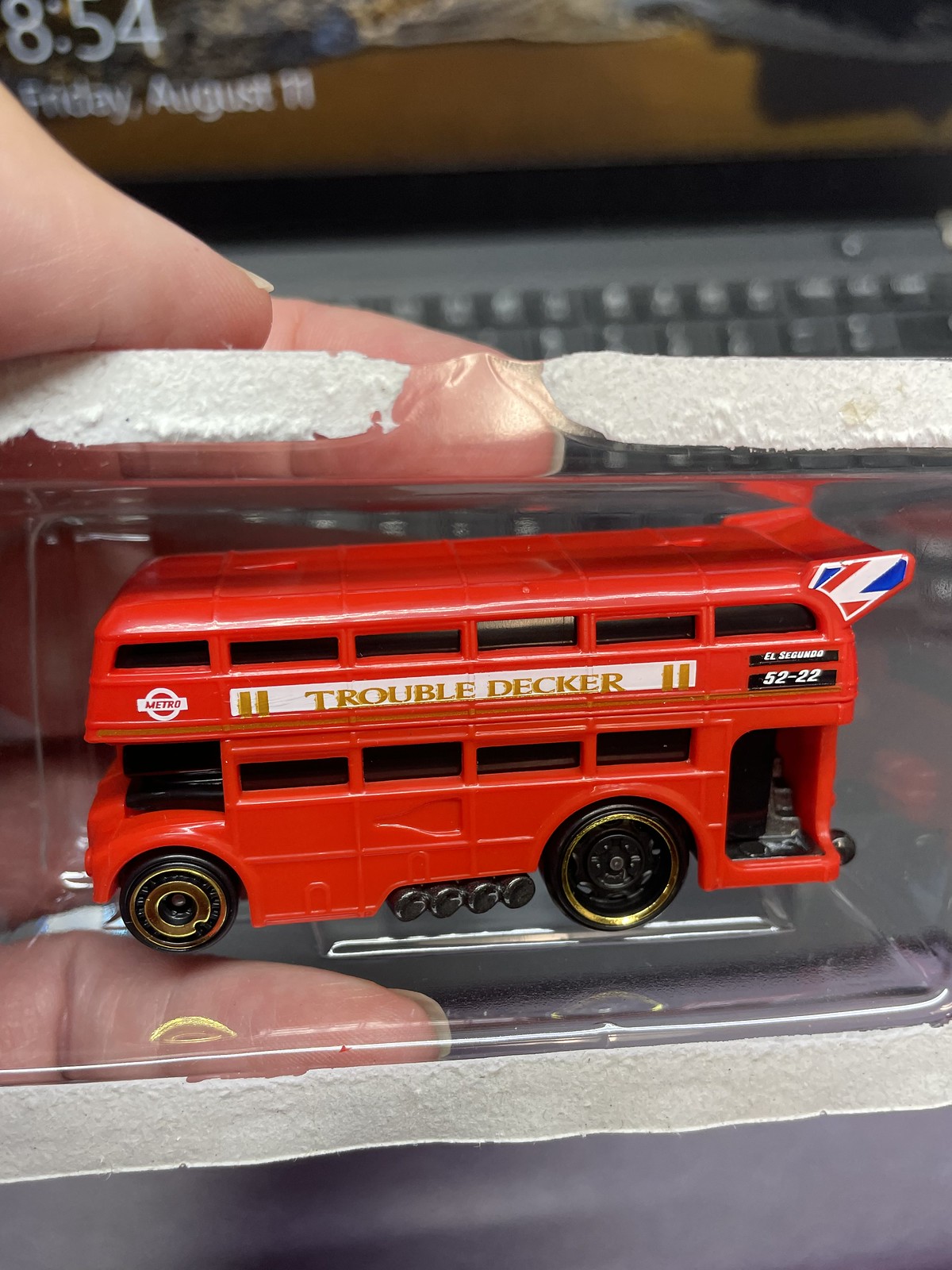The photograph is a close-up shot of a person's fingers holding a red, double-decker toy bus, which is encased in a clear plastic container. The bus, themed with the British flag on its spoiler, prominently displays the playful name "Troubledecker" along with the number 52-22. The wheels are black with golden rims. Behind the vividly detailed miniature, a laptop screen is visible, showing a beach wallpaper dated and timed as 8:54 AM, Friday, August 11th. The person appears to be displaying the bus, possibly suggesting it holds some value or significance.